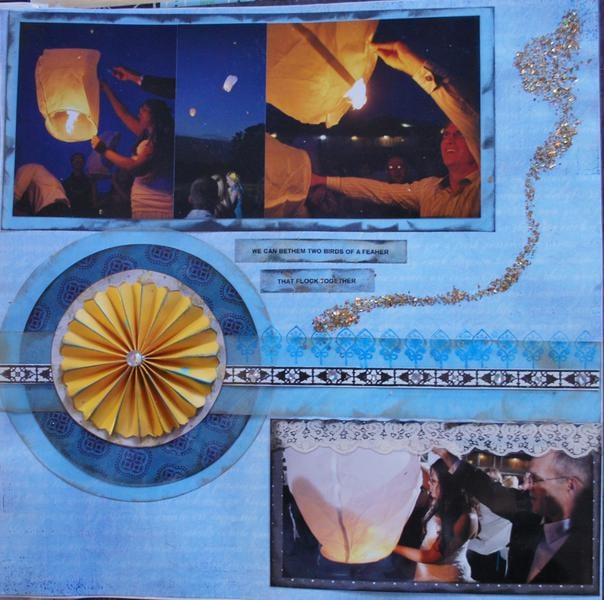The image appears to be a page from a scrapbook with a blue background, featuring multiple elements arranged in a collage-like manner. The top section of the layout includes a series of photographs showing people, outdoors at night, launching and holding balloons or kites. These balloons or kites seem equipped with a mechanism that emits fire, illuminating the night scene beautifully.

A prominent decorative element is a handmade paper flower with pleats, positioned on the left side of the image. At the heart of this yellow flower is a small, diamond-like white gem. Surrounding this flower is a streak of glitter, adding a touch of sparkle to the overall composition.

In the lower right-hand corner, there is a rectangular panel with a black background. This panel showcases a photograph of an older man and a woman. The man is on the right, and the woman is to his left, both involved in launching a white balloon, possibly symbolizing a traditional or festive event. This section also features lace details at the top and some writing underneath one of the upper images, though the text is partially obstructed and reads, "we can, we can, something, two birds of a feather that flock together."

A notable element tying the collage together is a black and white decorative line running horizontally across the image. This scrapbook page effectively combines personal photographs, handcrafted details, and textual elements to create a visually engaging and meaningful composition.